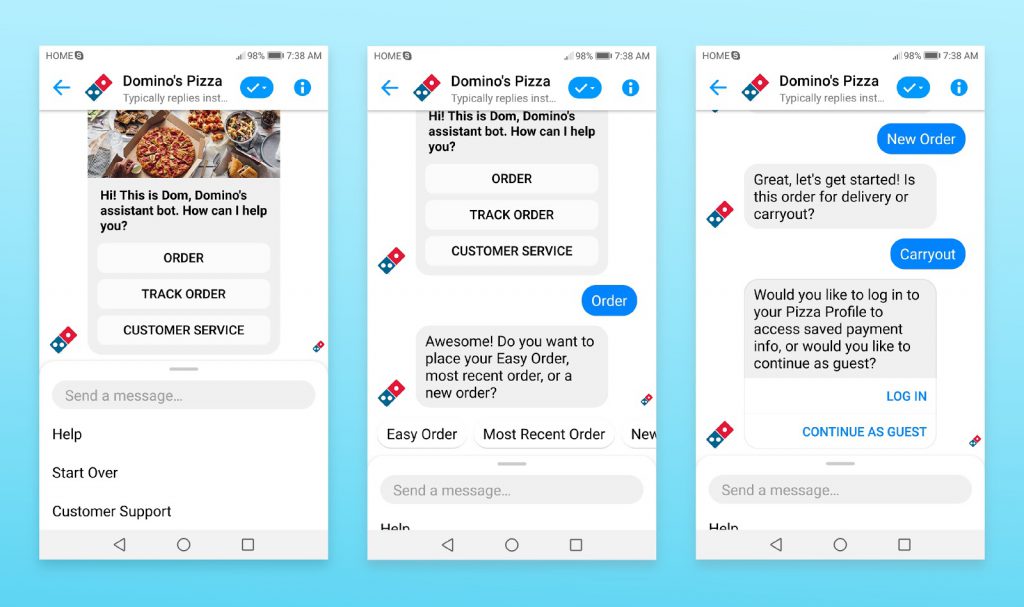The image depicts the Domino's Pizza website as viewed from three different smartphones, potentially the same model, but showing various stages of interaction with the site:

1. **Left Phone Screen**:
   - The top-left corner displays the time as 7:38 a.m., with icon indicators for signal strength and battery life next to it.
   - Centrally, the screen shows the Domino's Pizza logo. 
   - An arrow pointing left is on the left side, and a blue oval checkmark is on the right.
   - Below the logo, a message from Dom, Domino’s assistant bot, appears: "Hi, this is Dom, Domino's assistant bot. How can I help you?" 
   - Options listed for interaction include "Order Menu," "Track Order," and "Customer Service." 
   - At the bottom, there’s a text box labeled "Send a Message," followed by "Help," "Start Over," and "Customer Support."

2. **Middle Phone Screen**:
   - The format is similar to the left one, but with a response visible: "Awesome, do you want to place your easy order, most recent order, or a new order?"
   - Quick action buttons below read "Easy Order" and "Most Recent Order," with "New Order" partially cut off.
   - The text input area appears at the bottom.

3. **Right Phone Screen**:
   - This screen continues from where the middle one left off, showing the next step in placing a new order.
   - The bot’s message reads: "Great! Get started. Is this order for delivery or carryout?"
   - Options for "Login," "Continue as guest," and a message input area are present at the bottom, indicating ongoing interaction options.

Each screen detail provides a comprehensive look at the user experience of interacting with Domino's Pizza's online ordering system through their virtual assistant, Dom.